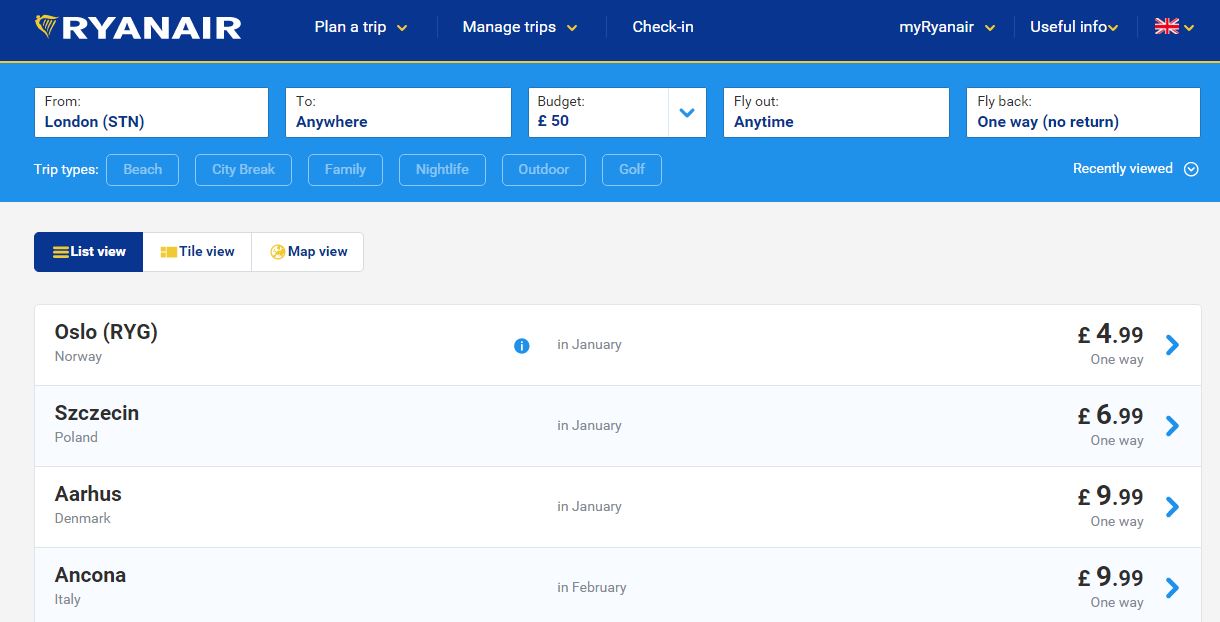The image showcases the Ryanair launch page, designed for the low-cost and budget-friendly European airline. The background of the page is a muted gray, with the distinctive Ryanair logo positioned in the upper left corner. The logo features a golden harp and the word "Ryanair" in bold, white, all-caps text.

Below the logo, there is a navigation menu with several options: "Plan a Trip," "Manage Trips," "Check-In," "My Ryanair," and "Useful Info." Each of these headings, excluding "Useful Info," features drop-down menus for further functionality. Positioned to the upper right, next to the navigation menu, is a Union Jack icon indicating that the language is set to English.

The main body of the page features a large, white search box for trip planning. Within this search box, users can input their departure location (e.g., London, STN), destination ("Anywhere"), budget (e.g., £50), and travel dates ("Fly out anytime," "One way, no return"). Just below the search box are categorized trip types including "Beach," "City Break," "Family," "Nightlife," and "Outdoor Golf," for users to refine their travel preferences.

To the right of the trip types, there is a "Recently Viewed" section. Below the main search area, the page transitions to a results section, which can be viewed in three formats: List View, Tile View, and Map View. Currently, List View is highlighted.

The List View showcases destinations like Oslo, Norway (RYG) for $4.99 one way in January; Szczecin, Poland for £6.99; Aarhus, Denmark for £9.99; and Kona, Italy for £9.99. All prices are for one-way tickets in January or February.

This detailed layout allows users to easily navigate the planning and booking process for their budget travels with Ryanair.